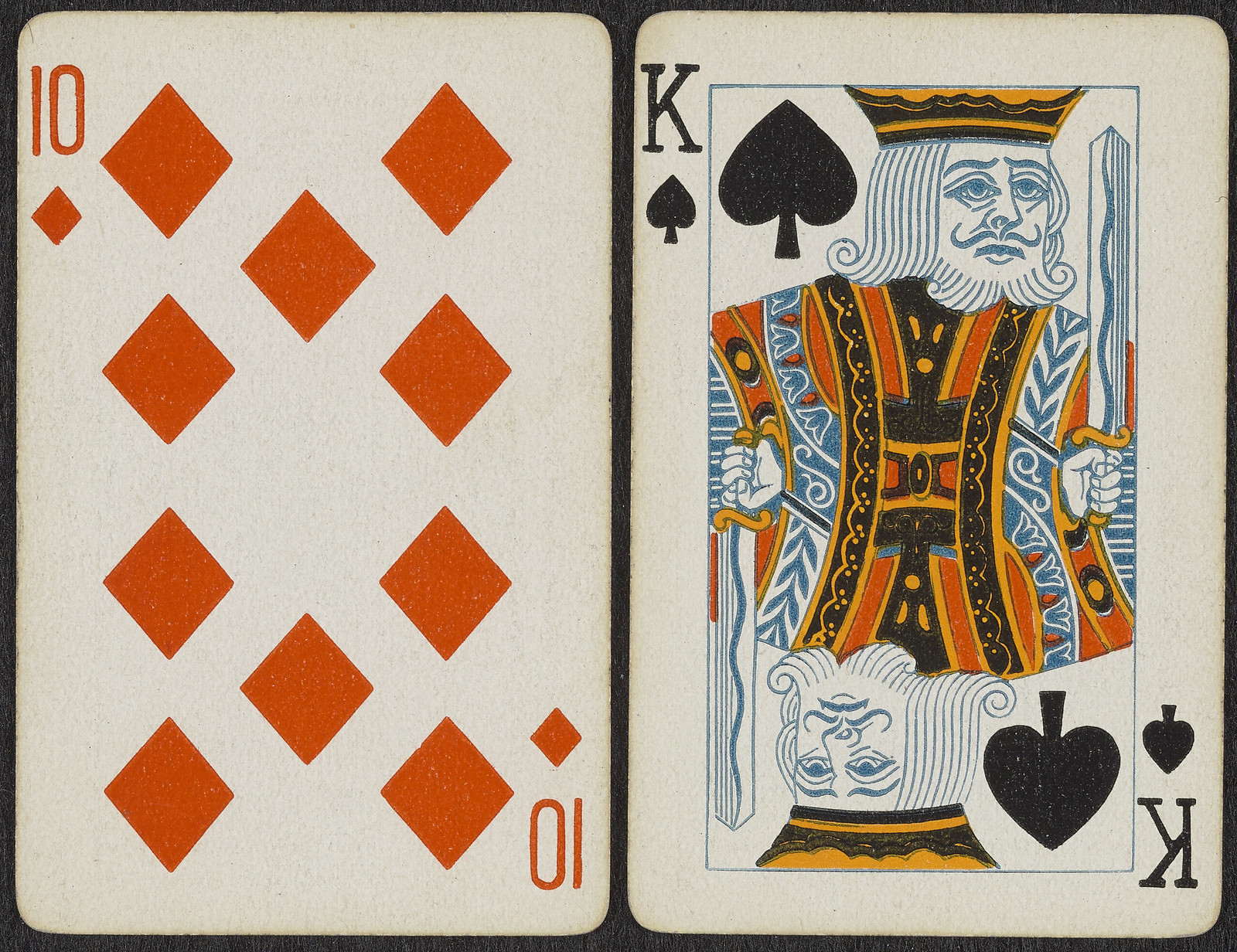This photograph features two well-worn playing cards, suggesting extensive use. On the left is the Ten of Diamonds, and on the right is the King of Spades. These cards have a classic, almost vintage appearance, reminiscent of decks commonly found in casinos or tucked away in a grandparent's drawer.

Both cards are displayed against a solid backdrop that appears to be either black or a very dark brown. The cards are positioned side-by-side with small gaps around the edges, giving each card its own space within the frame.

The King of Spades stands out due to its detailed and somewhat old-fashioned design. The intricately drawn king is adorned with a brown, red, and gold vest and a crown of similar hues. He holds a silver sword that features a gold handle and hand guard. This depiction captures the regal essence of a traditional deck of cards.

In contrast, the Ten of Diamonds is depicted in a more straightforward manner, featuring the standard layout of ten diamonds arranged symmetrically. The number ten is placed in the top left and bottom right corners, appearing both right-side up and upside-down to maintain visual consistency regardless of the card's orientation.